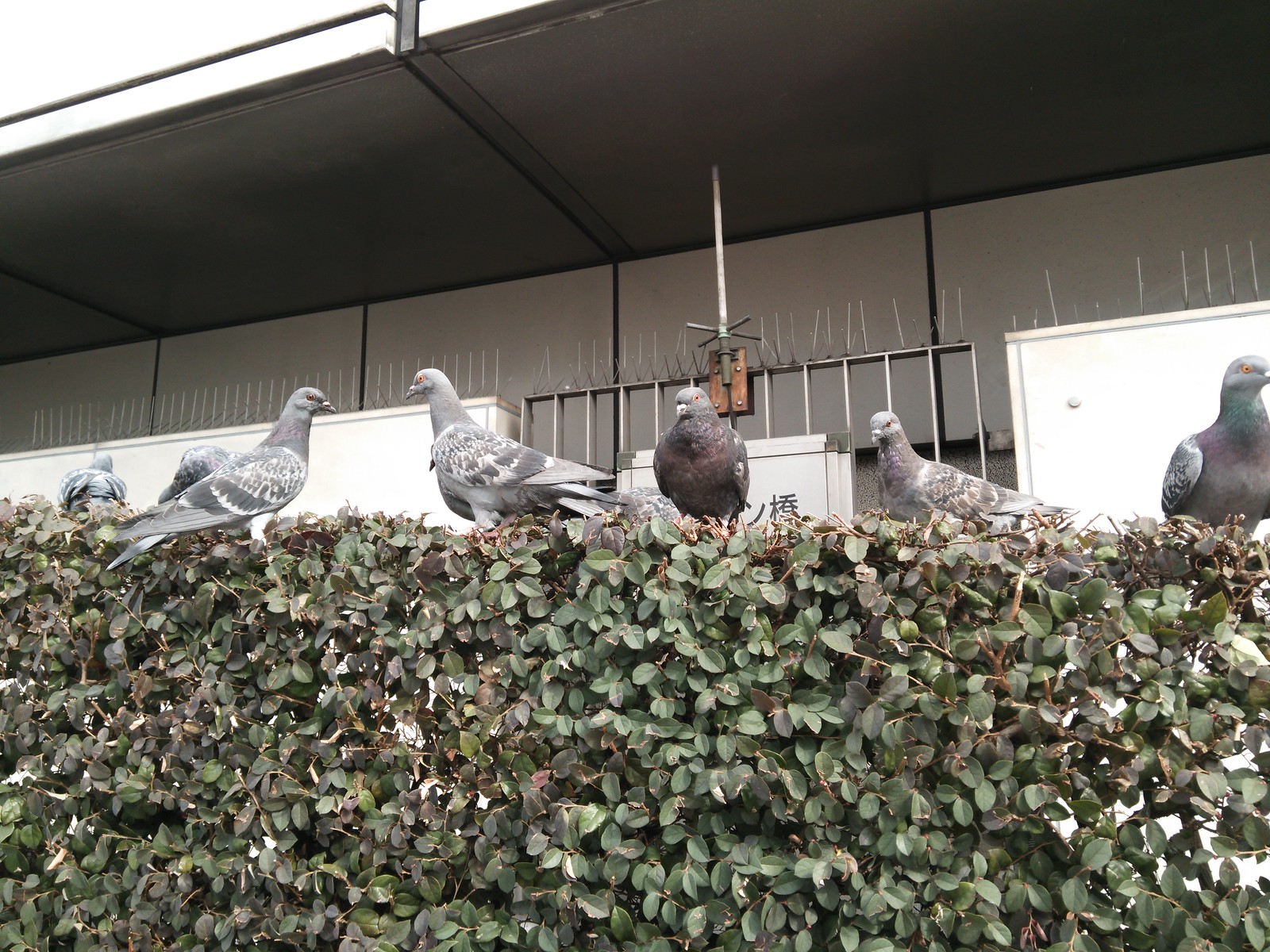This outdoor photograph captures a scene featuring a green hedgerow that stretches horizontally across the image, taking up about half of the composition. Perched atop the hedge are seven pigeons of various colors, some entirely gray with white accents, while others display strikingly colored plumage including red, pink, green, and black feathers particularly around their necks and wings. Behind the hedge, there's a metallic gate and a white wall adorned with Chinese writing. The structure in the background appears to be a large building, possibly an apartment building or a bar, with preformed panels and a roof overhang. Metal spikes are visible along the railing of the building, likely intended to deter pigeons. The scene is set during daytime, and the pigeons are depicted in various poses—some with their backs turned, others facing different directions, creating a dynamic and detailed composition.